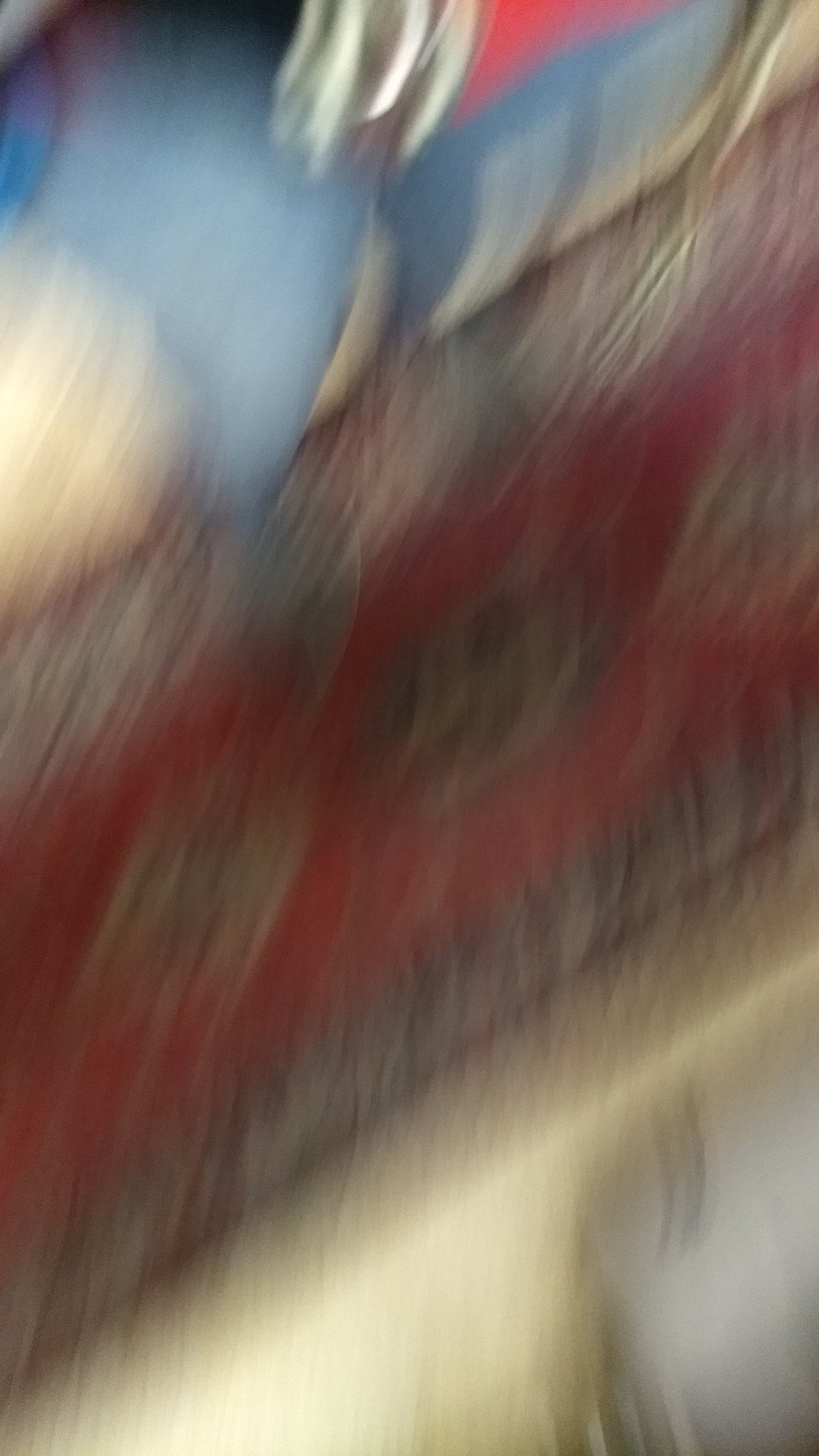The image is quite blurry, likely due to motion, and was taken vertically with a phone camera. In the foreground, there's a red throw rug or area rug with a brown trim and a pattern of circular shapes in cream and brown, extending across the center. At the top of the image, we see what appear to be cushions or pillows positioned against a couch or bed. These cushions have a mix of colors: white, blue, and some red. The background cushion, which appears larger and reddish-brown, contrasts with the smaller, cushiony blue ones in front of it. Additionally, there are some bold blanket or couch cushion patterns with large red circles and diagonal black lines. The top right and middle portion of the image might contain strands of long blonde hair, adding to the blur and complexity of the scene.